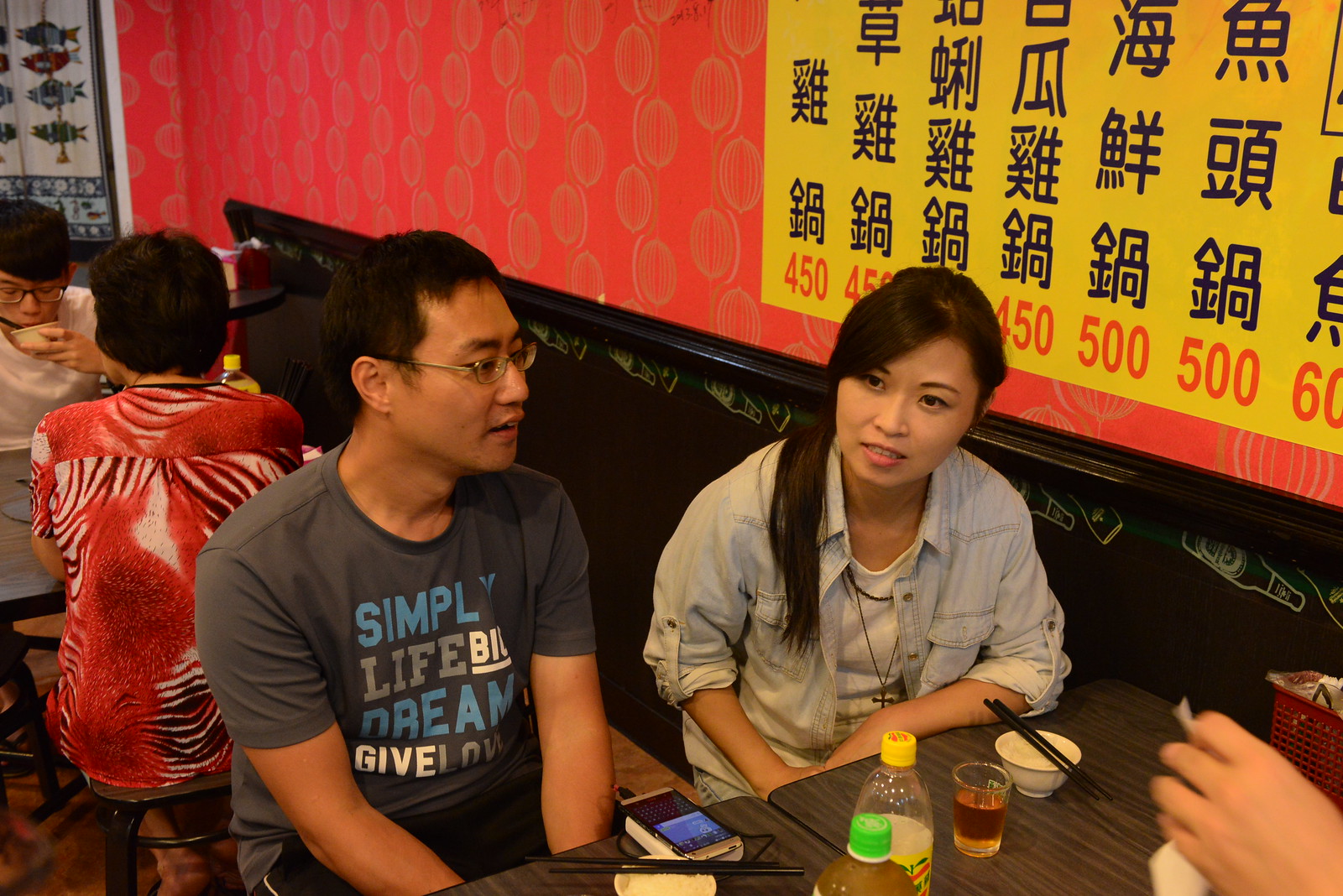In a cozy restaurant adorned with red wallpaper featuring gold-green circular patterns and black wooden paneling, several patrons are captured in a moment of dining. The setting suggests a Chinese restaurant, emphasized by a prominent yellow sign with Chinese script on the wall. The main focus is a young couple seated on the same side of a table. The man, with dark brown hair and wearing glasses, sports a gray shirt emblazoned with the phrases "Simply Life, Big Dream, Give Love.” The woman beside him, with long black hair, is dressed in a light blue shirt over a white t-shirt. They have finished their meal, as indicated by the bowls of rice and drinks on the table. Nearby, an older woman in a red blouse shares a meal with a younger man in glasses, adding to the lively yet intimate atmosphere of the restaurant.